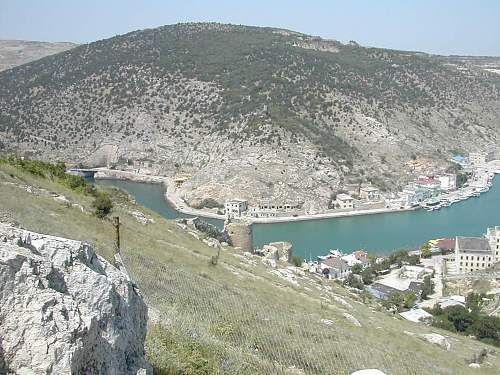This image captures an expansive view from a high vantage point on a hillside. In the foreground, a large rock or small boulder juts out from the left bottom corner, anchoring the scene. Below, the grassy hillside descends towards a small town or city nestled along a striking blue-green river. On the opposite riverbank, another small mountain rises, its slopes sparsely dotted with green bushes, small trees, and shrubs.

The town features a mix of homes, possibly hotels, and other buildings that hug the shoreline. There are distinctive structures such as a small building with multiple windows that could be a church or school, and nearby, a round structure resembling a lighthouse. The area also includes a parking lot and various residential and commercial buildings.

Looking higher up the mountain, patches of tan earth intersperse with greenery, leading towards the peak, which offers a stunning contrast against the light blue sky. A fenced area at the base of the mountain seems to denote property boundaries, adding a human touch to this scenic landscape.